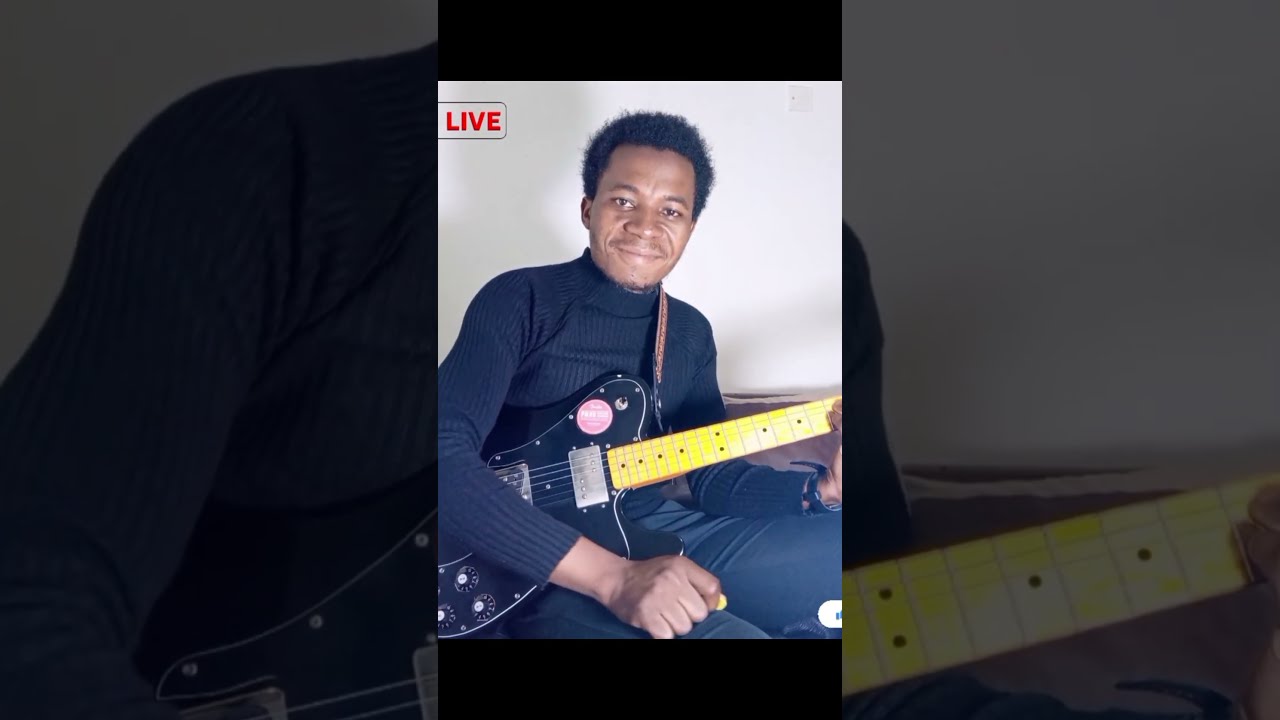The image is a rectangular, horizontal composition divided into three frames. The central frame features a detailed photograph of a seated Black man wearing a black turtleneck shirt and dark pants. He is holding a black electric guitar with a yellow neck, which is secured with a strap over his shoulder. The man's dark, curly hair and short hairstyle are visible as he looks directly into the camera, his right hand closed in a fist resting on his thigh. The peripheral frames on either side are grayed out and appear to be blown-up and low-exposure sections of the central photograph, adding a dark, abstract contrast. 

A light source from the right casts a shadow on the left, where a red rectangular box with the word "LIVE" in uppercase white letters appears in the upper left corner of the central frame. This could indicate a live performance or possibly an album cover.